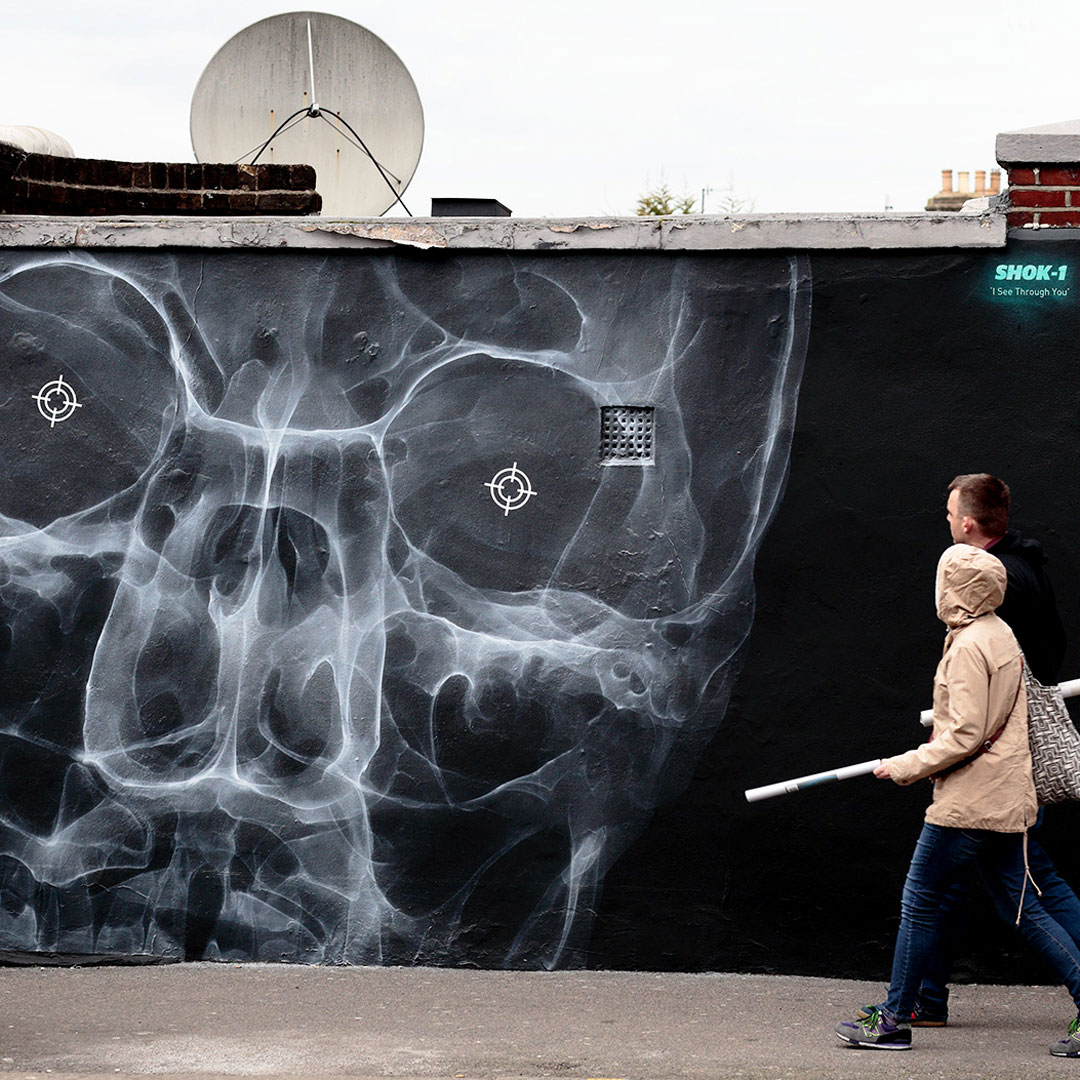The photograph captures a striking mural painted on a black wall, predominantly featuring an x-ray depiction of a human skull. This skull mural is adorned with eye sockets that contain white target crosshairs, giving it a hauntingly precise look. Above the mural, a ragged cement top of the wall is visible, crowned by a satellite dish. The graffiti art is further accentuated by the inscription "Shock 1 I see through you" in green neon paint. Additionally, two individuals – a man and a woman – are walking mid-stride on a gravelly sidewalk in front of the mural. The man is dressed in black, blending seamlessly with the mural's dark background, while the woman wears jeans and a light brown jacket. The detailed combination of art and urban life adds depth to this visually captivating scene.